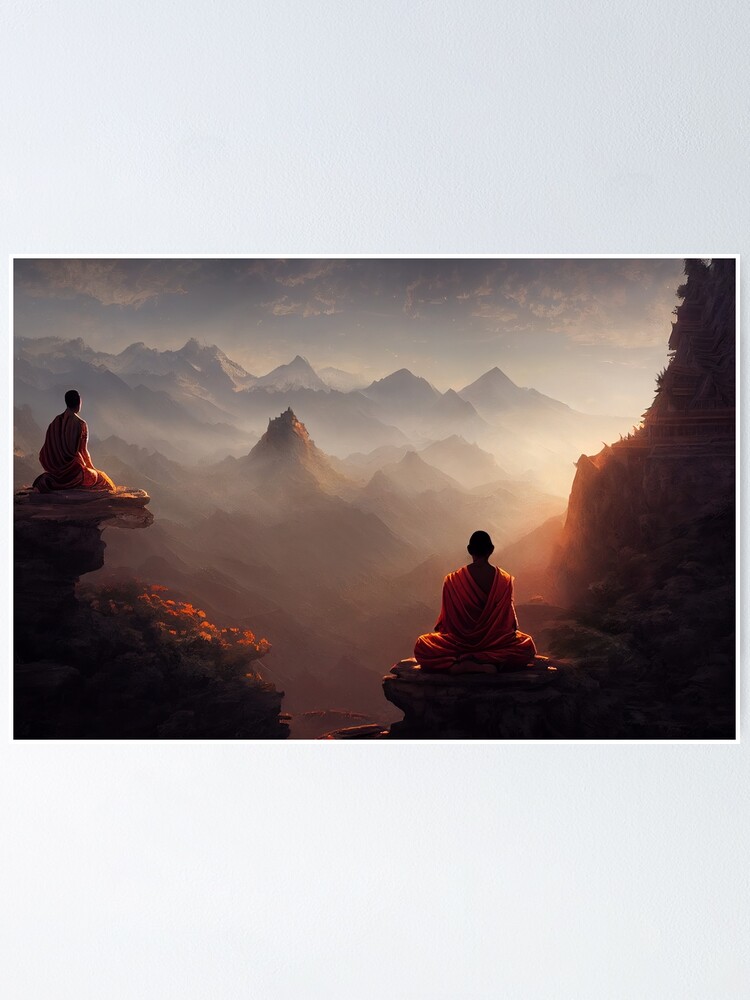In this striking photorealistic image, two Buddhist monks, adorned in saffron robes and with short hair, are seen perched atop rocky mountain outcroppings, absorbed in meditation. One monk is positioned closer to the bottom right, facing away from us, while the other, in the top left, is in a three-quarters view looking off to the right. The monks are set against an expansive, jagged mountainous landscape that stretches far into the distance, with peaks gradually fading into shades of gray as they recede. The foreground mountains exhibit an orange glow, a hint of green, and interspersed trees, creating a striking contrast with the misty, fog-like atmosphere enveloping the mid-ground. Above, a sky filled with partially grayed-out white clouds suggests either dawn or dusk, with sunlight casting an ethereal glow from the right side, illuminating a temple. This temple, intricately built into the mountainside, towers vertically and appears as a dark, backlit silhouette on the far right. The overall composition conjures a peaceful, almost mystical ambiance against the dramatic and detailed landscape.